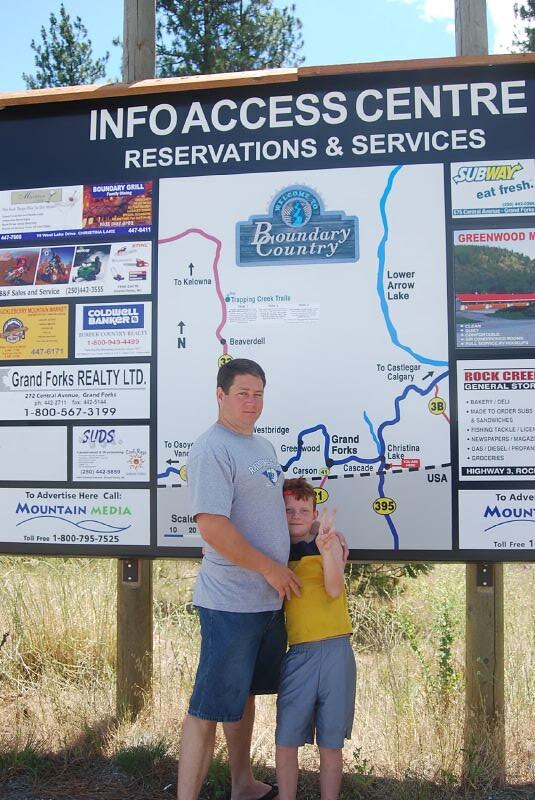In this outdoor daytime photograph taken in portrait mode, we see two Caucasian males - an older adult, likely in his mid-30s, and a young boy, around 10 years old. They are standing on tall, light brown grass near the side of a road in front of an information sign supported by two vertical wooden posts. The backdrop includes some trees and a bright blue sky with a few white clouds.

The older adult male has short dark brown hair and is dressed in a light gray, short-sleeved T-shirt adorned with a logo, along with blue shorts. His body is slightly angled to the right, but he looks directly at the camera with a warm expression. Snuggled into his stomach area stands the young boy with reddish hair. The boy is wearing a yellow short-sleeved shirt, light blue shorts, and a red headband, which holds back his fiery hair. He has a playful demeanor, raising his left hand to flash a peace sign at the camera.

Behind them is a large board with important local information. The top of the board has a dark blue border with white text, reading "Info Access Center, Reservations and Services," and below it features a map labeled "Boundary Country," detailing areas like Lower Arrow Lake, Castlegar, Calgary, and Grand Forks. Surrounding the central map are various advertisements from local businesses such as Subway and Coldwell Banker. The scene captures a moment of casual, friendly interaction against a backdrop of informational and regional details, embodying the essence of their location.